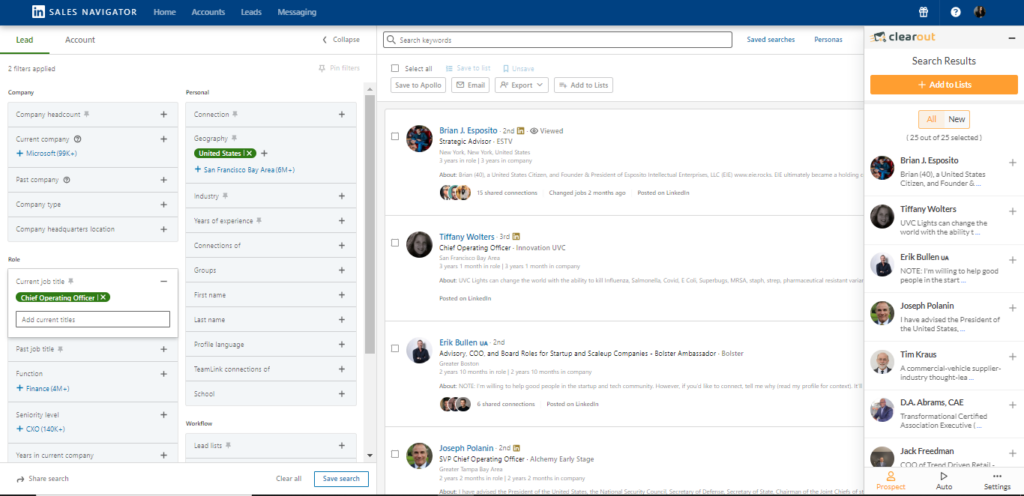The image depicts a user interface screen displaying various sections and features typically found in a business and networking platform. The prominent sections listed on the left-hand side of the interface include Home, Accounts, Leads, Messaging, Gift Cards, Lead, Account, Class, Search Keywords, Save Searches, Personas, and Clear Out. 

On the right-hand side, there's a column displaying further details and a row highlighting additional options and settings. The Settings menu features clickable profiles, such as Brian J. Espinosa and Tiffany Walters, who hold the title of Chief Officer.

Other components visible in the interface include Connections, categorized by Geography, Industry, and User Experience. Users can manage their Connections on Groups, viewing details about First Time and Last Time interactions, and can filter professionals by their team or seniority level. Further tools provided include a Hashtag to Know section and Function-specific filters. The interface offers a comprehensive and organized layout to streamline user experience and enhance professional networking efficiency.